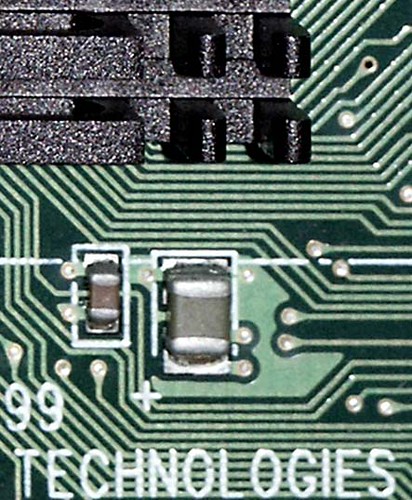This image is a close-up shot of a circuit board, possibly the backside, showcasing the intricate details of its design. The background is predominantly green with various shades of lighter green lines that create a network of intersecting connections resembling highways or roads. Prominent solder points are visible, especially around two rectangular components: one larger and reddish with white caps, and a smaller adjacent one featuring similar colors. There is also a noticeable plus symbol indicative of a positive connection. The upper portion of the image presents a grayish-black area with four components akin to memory cards or SIM cards, blending into the green circuitry. The text "99 Technologies" is prominently displayed in white at the bottom, along with a plus symbol and the number 99, adding a polished finish to this detailed electronic masterpiece.